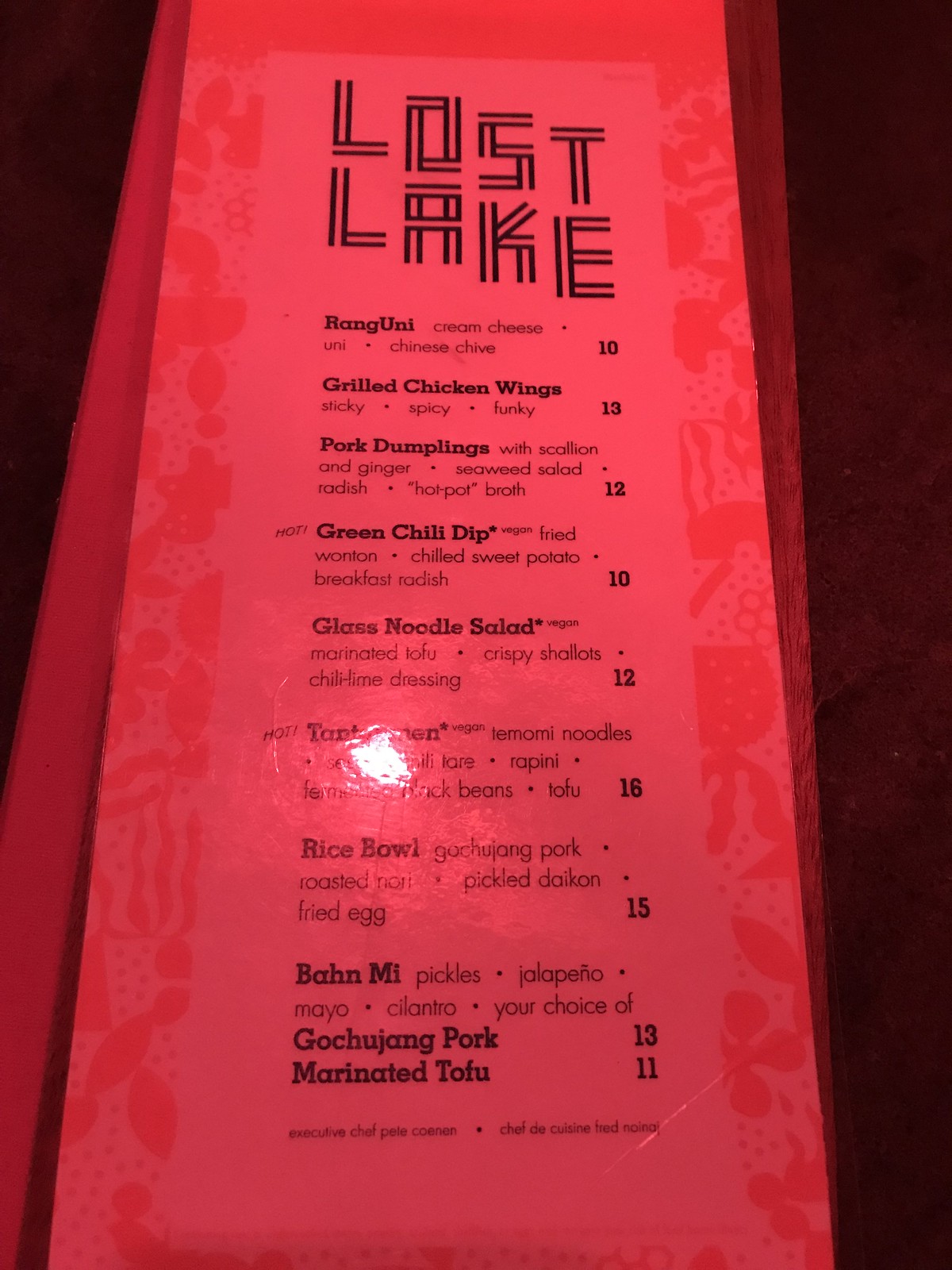The photograph captures a glossy menu set against a beautifully vivid reddish-pink background, bordered by intricate floral designs in deeper shades of red and pink. Reflection from a light source, likely from above or behind the camera, creates a shiny highlight across the lower half of the menu. 

The menu’s text is clearly displayed, headlined with "Lost Lake." It lists an array of tantalizing items: 
- Rang Uni
- Chinese Chive with Cream Cheese
- Grilled Chicken Wings (described as sticky, spicy, and funky)
- Pork Dumplings with Scallion and Ginger
- Seaweed Salad with Radish
- Hot Pot with Broth
- Green Chili Dip
- Glass Noodle Salad
- Rice Bowl
- Balmy Pickles
- Jalapeno Mayo and Cilantro with a choice of Pork or Tofu.

Each item is accompanied by numbers, presumably indicating their prices: 10, 13, 12, 10, 12, 18, 16, 15, 13, and 11, respectively. The header announces "Lost Lake," and near the bottom, the title "Executive Chef" is visible, though the name is not legible. The visually striking menu sets an inviting tone for this establishment known as Lost Lake.